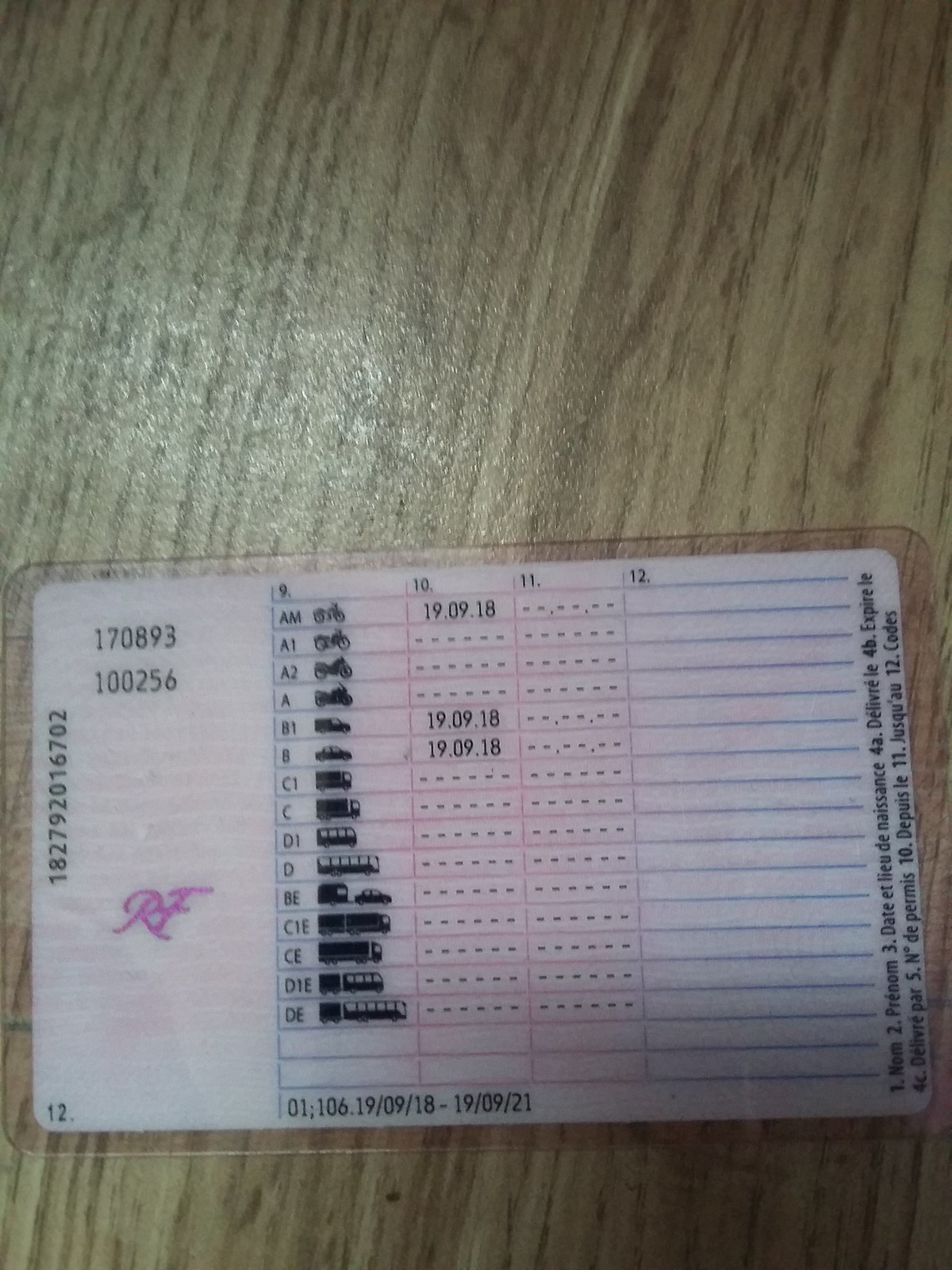The image depicts a laminated plastic card placed on a wooden table, featuring a detailed grid of rows and columns. In pink letters on the side, the card is labelled "RF," and a series of numbers is present on the left side. The primary table consists of columns numbered 9, 10, 11, and 12. The first column includes a series of letters referencing various vehicle types in a foreign language, likely French. These classifications are as follows: AM, K1, A2, A, B1, B, C1, C, D1, D, BE, C1E, CE, D1E, and DE. Beside these letters in column 9 are small images depicting motorcycles, cars, buses, and other vehicles, aligned with their respective classifications. Column 10 contains additional numbers, while columns 11 and 12 remain blank. On the right side of the card, some text appears sideways, though it is illegible. At the bottom, another set of numbers can be seen. This card serves to classify different types of vehicles according to a specific foreign system, indicating the various permissible vehicle categories for different licenses.